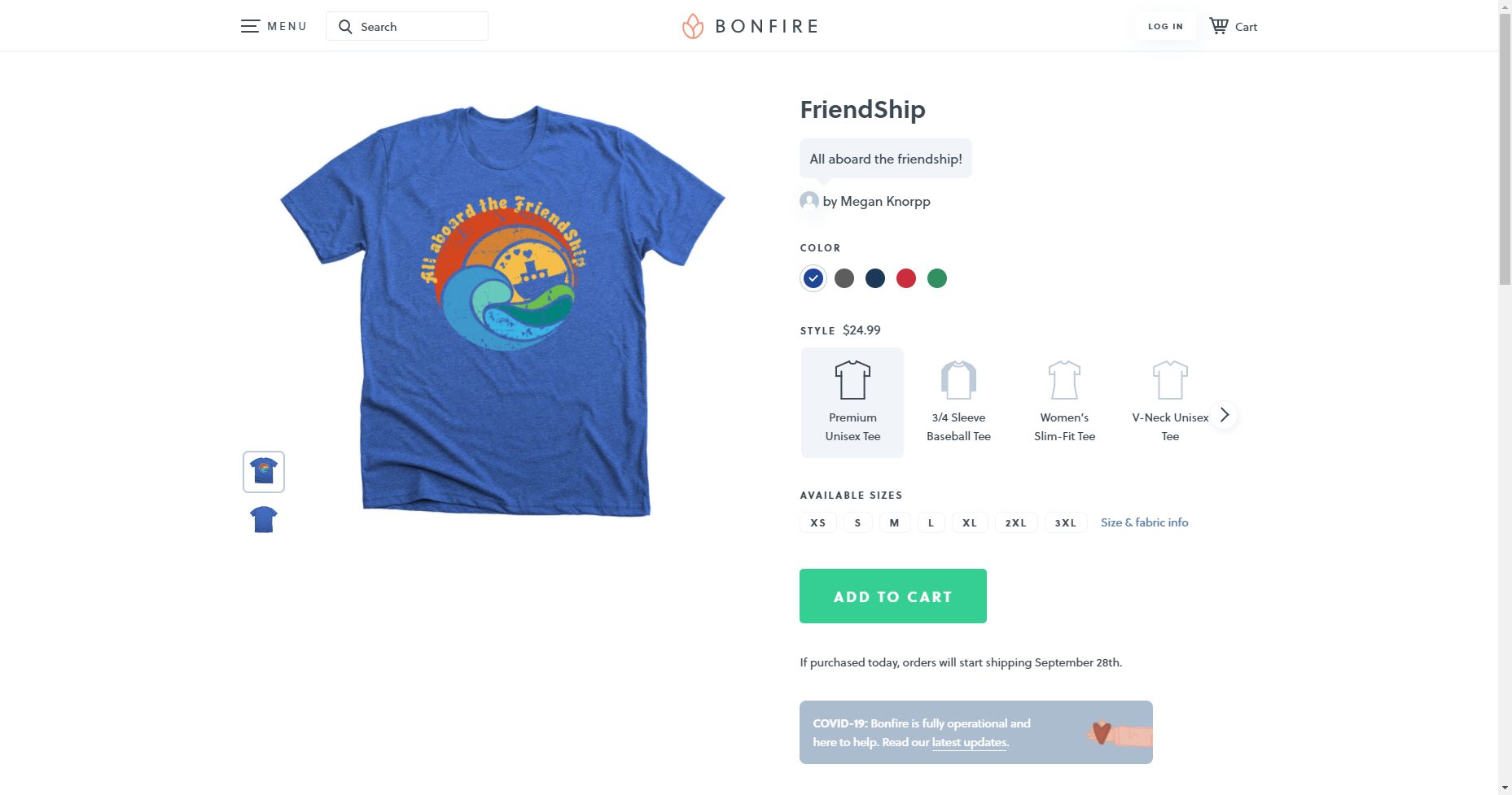Certainly! Here’s a detailed and polished caption:

---

The screen displays an online ordering site named Bonfire, identifiable by its logo and name prominently placed at the top center. The focal point of the page is a blue T-shirt featuring a circular design. At the top of the circle, arcing from left to right, the phrase "All Aboard the Friendship" is inscribed in gold lettering. Below this text, the circular design transitions through bands of red, pale orange, and yellow, featuring a blue ship at its center. Beneath the ship, blue, green, and pale blue waves are depicted, all encompassed within the circular motif.

To the left of the main image are two smaller thumbnails of the T-shirt, allowing views of both the front and back. The upper-left corner features a menu icon represented by three horizontal lines, a magnifying glass beside a search bar, and the entire backdrop of the page is white. On the right side of the screen, the T-shirt description reads, "Friendship, All Aboard the Friendship by Megan Knorp."

The T-shirt is available in various colors: blue, gray, black, red, and green (displayed from left to right). It also offers an array of size options and styles including Premium, Unisex, Three-Quarter Sleeve, Women's Slim Fit, and V-neck Unisex. Sizes range from XS to 3XL. Beneath the size and style options is a green rectangle button labeled "Add to Cart." A shopping cart icon is located at the upper right of the screen for easy access to the checkout process.

The T-shirt in the main image appears slightly wrinkled, laid out flat with its short sleeves sticking out on either side. This standard short-sleeved T-shirt is presented along with various styling options, ensuring a customizable shopping experience.